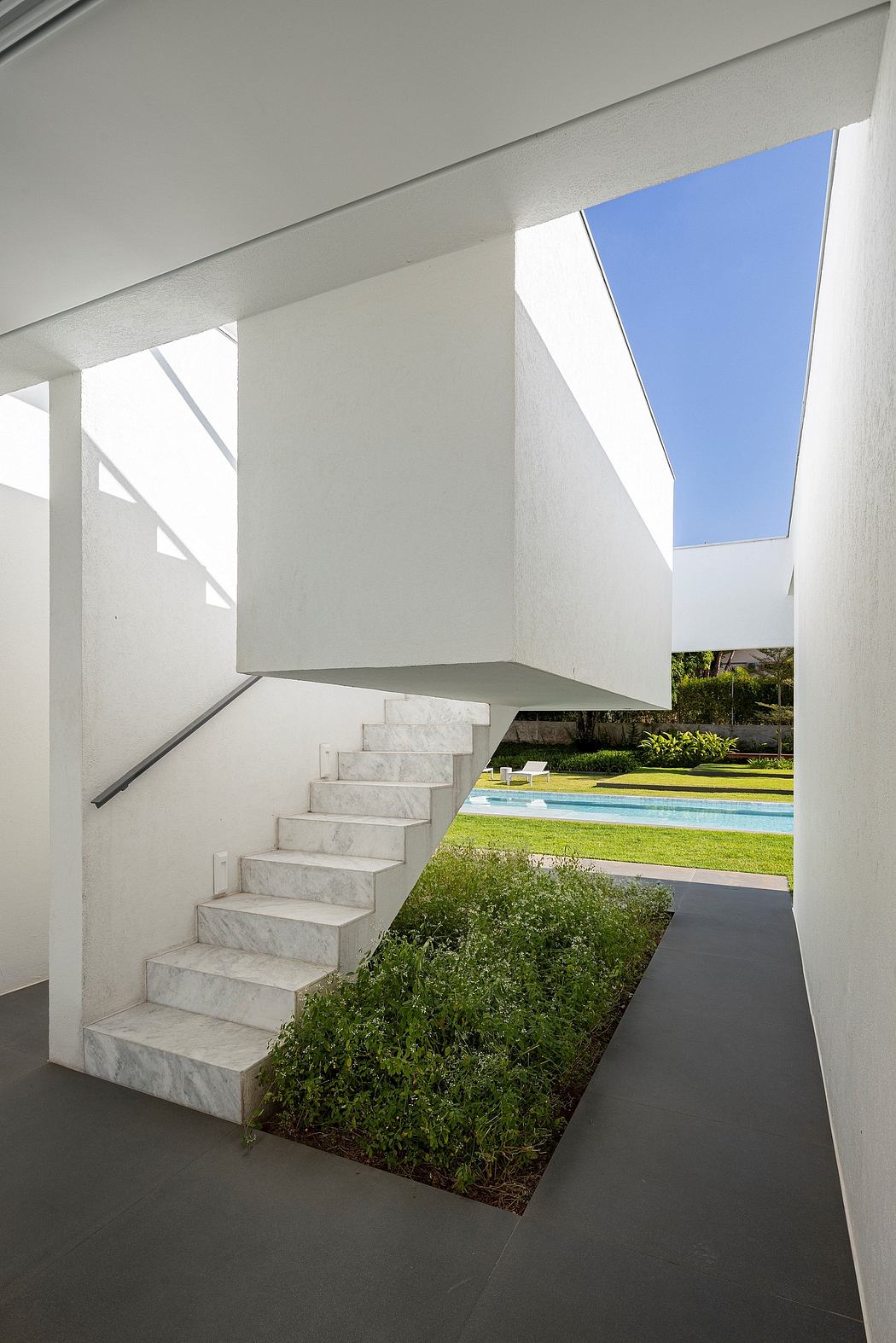The image depicts a modern, minimalistic mansion situated in a likely secluded, sunny, desert-like area. The photograph is taken from within a white-tiled corridor framed by two white walls, suggesting a main entrance or an alcove. On the right, a stark white wall contrasts with the dark gray tiles on the floor. To the left, there is a prominent staircase with a marbled pattern on each of its ten steps, climbing towards the second story of the structure. This staircase has no railing on the right side but is bordered by a half-wall handrail on the left. Adjacent to the stairs, there's a small but overgrown patch of grass or shrubs. Beyond the corridor, the backyard boasts a rectangular swimming pool accompanied by a lawn chair, and is surrounded by more grass and low landscaping plants. The clear blue sky above accentuates the airy, open feel of the property.